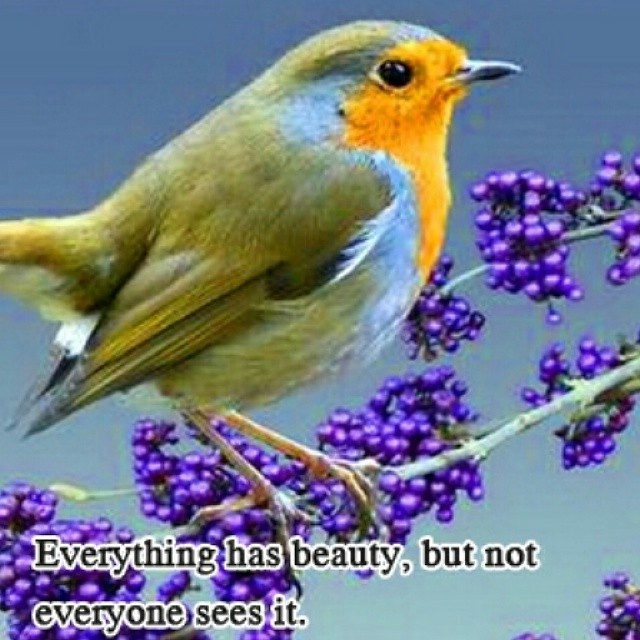The image features a small, vividly colored bird perched on a white twig, surrounded by smaller branches laden with small purple berries. The bird, resembling a budgie or swallow, has a striking appearance with a yellow breast and face, transitioning to blue on its head and then green on its wings. Its chest below the yellow is tinged with another shade of blue. The bird’s eyes and beak are black, giving it a distinct, detailed profile as it looks to the right of the frame. The background is a solid blue, suggesting it's set high up in the sky, creating a dreamy, almost surreal ambiance. At the bottom of the image, a quote in black font with a white border around each letter states, “Everything has beauty, but not everyone sees it.” This quote underscores the picture’s artistic and thoughtful nature, making it a visually and emotionally appealing creation, likely intended for sharing on social media.